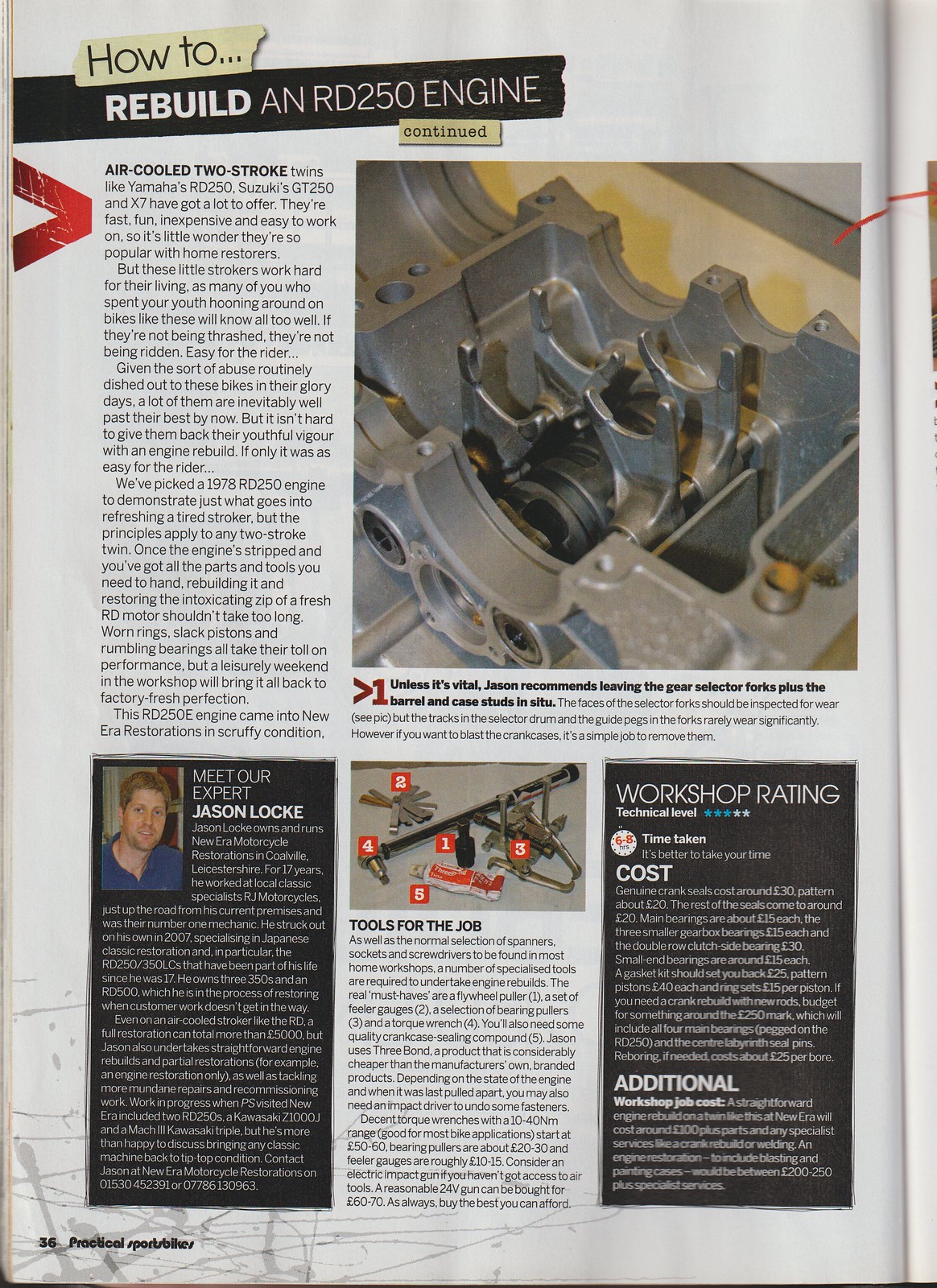The magazine article on page 36 of Practical Sports Bikes is titled "How to Rebuild an RD250 Engine Continued," prominently displayed in a yellow box with black text. The article discusses the appeal of air-cooled two-stroke twins like Yamaha's RD250 and Suzuki's GT250 and X7, describing them as fast, fun, inexpensive, and easy to work on, which makes them popular among home restorers.

A detailed close-up photograph on the right side of the page showcases the internals of a disassembled motorcycle engine, offering insight into where the pistons fit. The caption below this image advises on the maintenance of gear selector forks and other components, with expert recommendations from Jason Locke. Essential tips, such as inspecting the faces of the selector forks and noting that the guide pegs in the forks rarely wear significantly, are included.

The bottom left section features a "Meet Our Expert" profile of Jason Locke, complete with a small photo of him dressed in a blue shirt, sporting blonde hair, and a brief biography. Adjacent to this profile at the bottom center, a subtitle reads "Tools for the Job," accompanied by a photo of various tools labeled with numbers. Below this photo, there is descriptive text explaining the use of these numbered tools.

On the bottom right, the article provides a "Workshop Rating," listing the technical level, time taken (six to eight hours), cost breakdown, and additional job costs. The overall rating of the workshop, suggested by stars, is also noted here, guiding readers on what to expect from undertaking the repair.